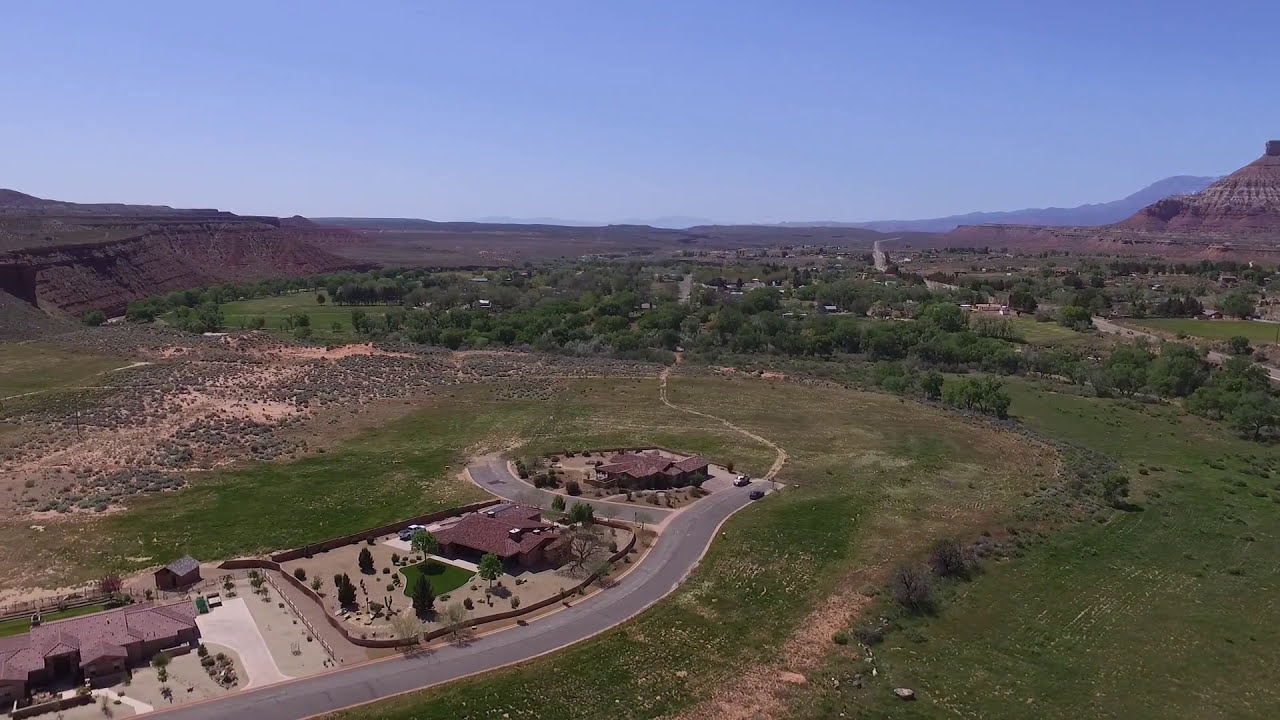The image is a bird's-eye view of a large, open grassy field bordered by steep drop-offs, almost cliff-like, on both sides, extending into a forested region. Cutting through the bottom left corner to the center of the image is a gray paved road that transitions from a curved dirt path. This road leads to three large brown houses, possibly mansion-sized, surrounded by gray gravel. Other elements in the photograph include green trees with lush, fluffy treetops, and sparse green bushes scattered across the surrounding properties. Beyond the houses and grassy field, there is a desert landscape with rocky formations, with a brown rocky hill on the left and extending to the horizon on the right. The sky above is expansive, light blue, and cloudless, with a slightly hazy appearance, and there are distant silhouettes of mountains.